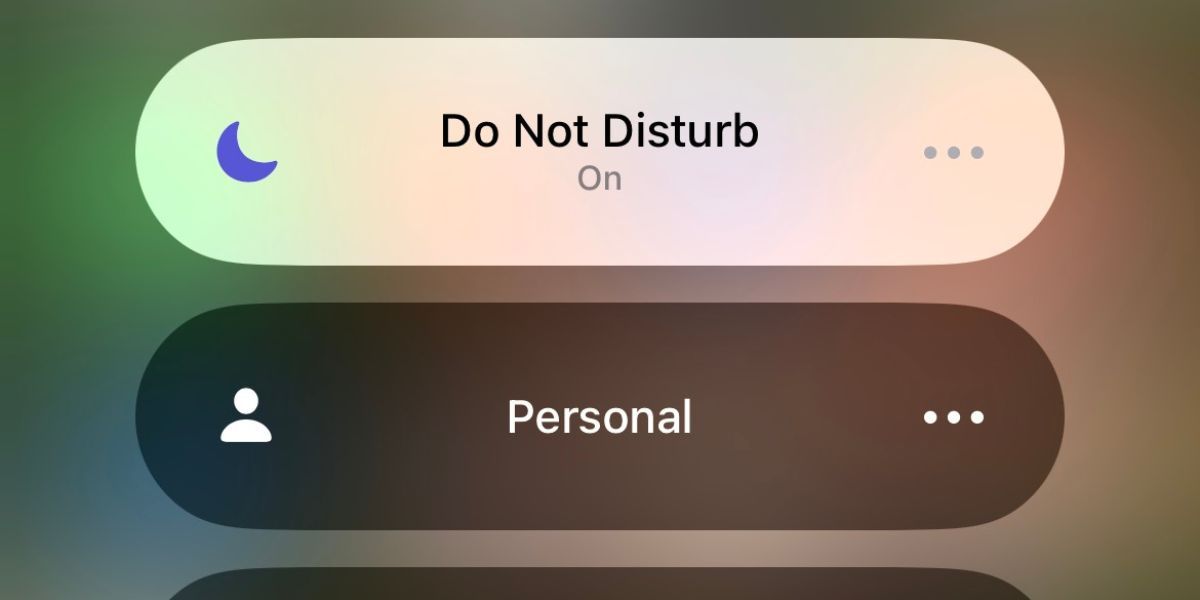**Close-Up of Smartphone Interface Featuring 'Do Not Disturb' and 'Personal' Buttons**

This closely framed image captures two primary buttons on a smartphone, exhibiting a vivid spectrum of background colors that are artfully blurred. In the center, the dominant feature is the 'Do Not Disturb' button, prominently displaying the black text "Do Not Disturb" at its center. Adjacent to this text on the left side, a delicate purple crescent moon icon subtly reinforces the function of the button.

Beneath the 'Do Not Disturb' button is the 'Personal' button, which is distinctly brown. The button's label, "Personal," is neatly centered and rendered in clean white font.

The background provides a gradient of colors, adding to the visual appeal without distracting from the main elements. Starting from the left, the hue begins with a green tint, which transitions into a tan shade towards the right. A touch of blue is visible at the bottom left corner, while the bottom right corner blends greenish and blackish tones.

The overall composition is a harmonious mix of utility and aesthetics, effectively highlighting the interface elements against a softly blended palette of colors.